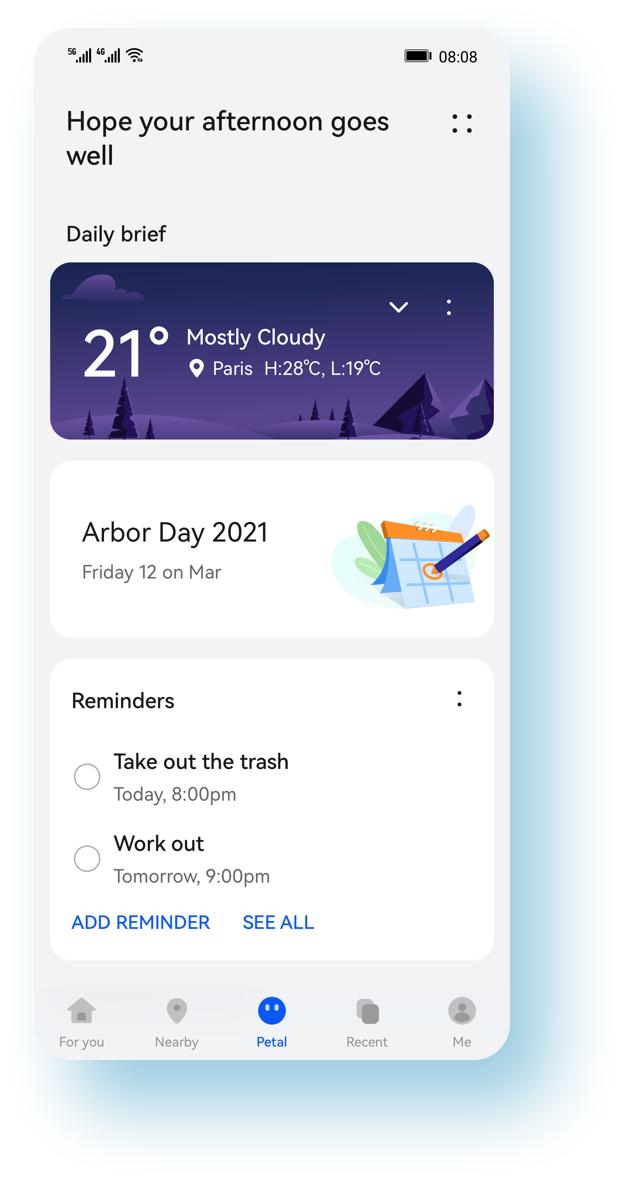The image portrays a smartphone screen displaying a mock-up of a notification panel with an exaggerated and unusually large sky-blue drop shadow. In the top section of the screen, service indicators show 5G and 4G bars along with Wi-Fi signal strength and a fully charged battery, while the time is displayed as 08:08.

The main section of the notification panel features a friendly message, "Hope your afternoon goes well," followed by a "Daily Brief." The brief includes a weather update for Paris, indicating a temperature of 21 degrees Celsius and mostly cloudy skies, with a high of 28 degrees Celsius and a low of 19 degrees Celsius. Accompanying this information is a graphic depicting a nighttime scene with purple hues, featuring pine trees on a snowy mountaintop.

Below the weather update, an entry marks "Arbor Day 2021," occurring on Friday the 12th of March, illustrated with a calendar graphic of a purple pencil marking a date. Further down, the "Reminders" section lists two tasks: "Take out the trash today at 8 p.m." and "Work out tomorrow at 9 p.m." Blue text options below these reminders allow the user to "Add a reminder" or "See all."

At the bottom of the screen, a navigation menu includes tabs labeled "You," "Nearby," "Petal," "Recent," and "Me." The app's name might be "Petal," though this is not confirmed. The most striking element of the image is the oversized drop shadow casting a bold sky-blue hue, making the mock-up appear surreal.